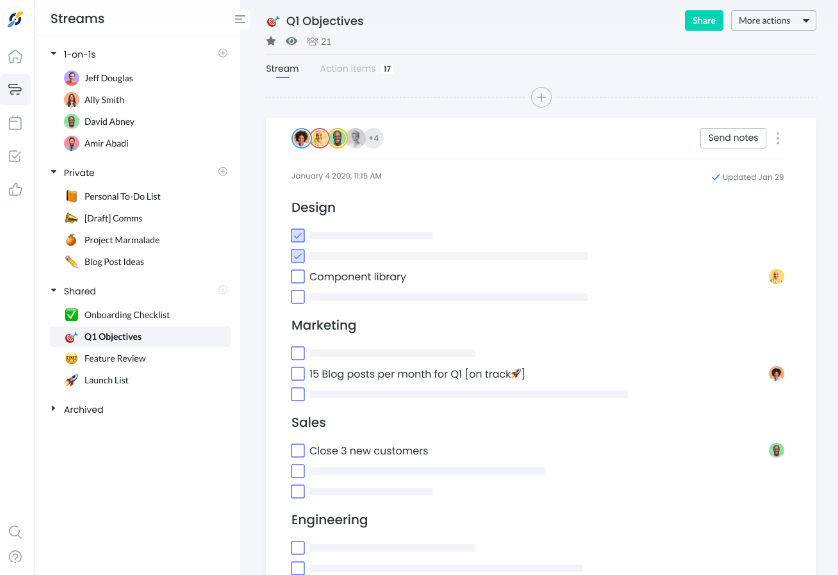### Detailed Caption for the Image

The image has a gray background and prominently features the Q1 objectives. Key visual elements include a star, an eye icon, and a number "21" next to an alarm clock symbol. There is a green rectangle labeled "Share" with additional options for "More Actions," "Stream," and "Action Item." This section also shows a "+17" indicator.

In the image, there are four profile pictures, along with a circle displaying "+4," indicating more participants. Other icons include "Send Notes" and three vertical dots for additional menu options. 

Below these elements, the image displays a timestamp "January 4, 2020, 11:15 AM" and notes an update on "January 29th" with a checkmark. The objectives listed are "Design," which has a checkmark next to it, indicative of completion. Another checked-off item is "Component Library." Additionally, marketing objectives include a line-item goal of "15 blog posts per month for Q1," marked with "On Track" enclosed in brackets and a rocket ship icon.

Sales objectives are described next, with a goal to "Close three new customers," followed by two lines under "Engineering." 

On the far left of the image, there are categories labeled "Streams, One-on-Ones, Private, Shared, and Archived," providing sections for organized views.